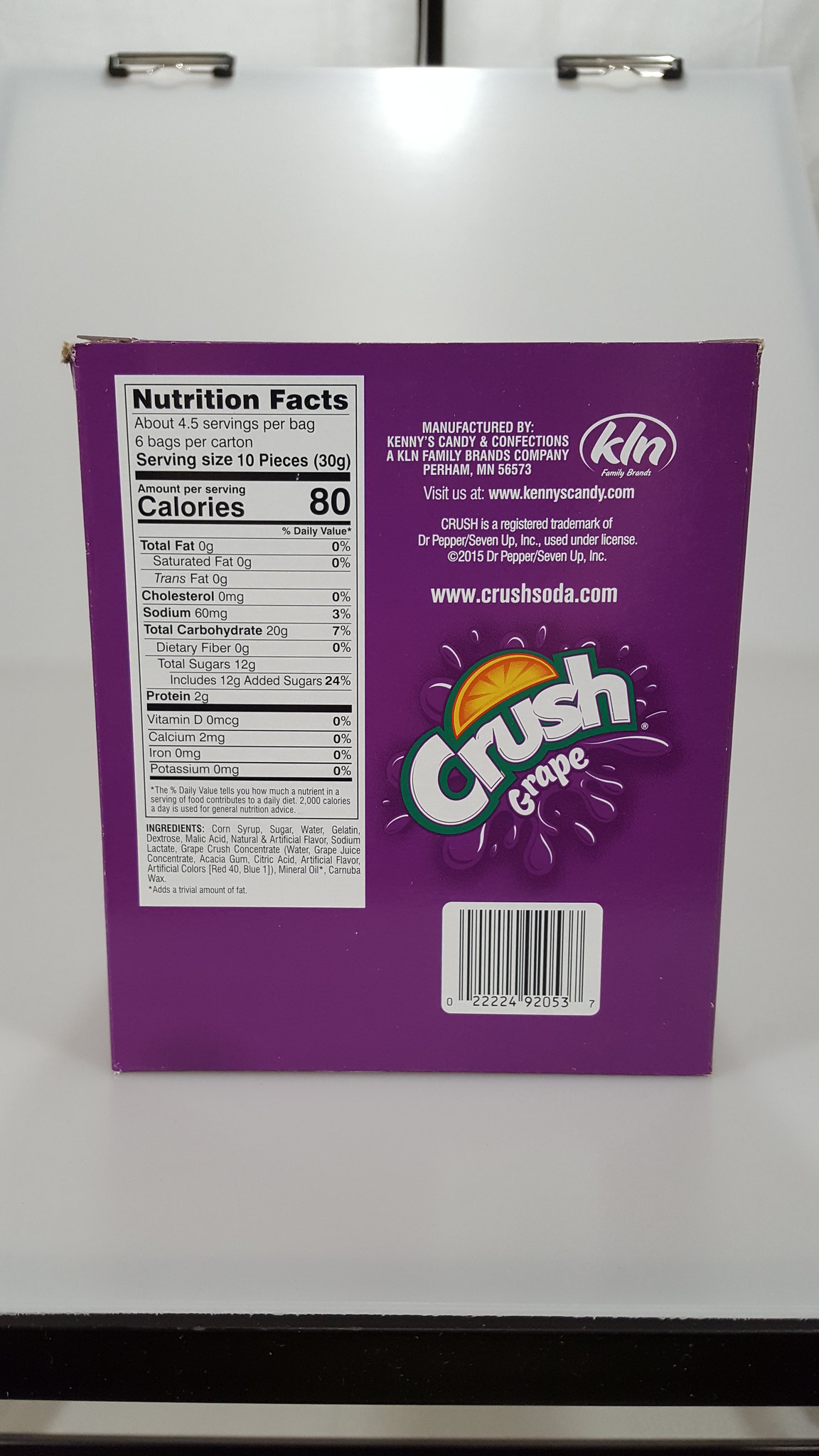This is a detailed photograph of the backside of a large purple carton, prominently featuring the Crush Grape soda brand. The carton is set up on a white background, presumably a whiteboard, with two clips visible at the top edges. The box itself has fraying on the top left corner. On the left side of the carton, there is a white label with "Nutrition Facts" in bold black letters. Underneath, it details that there are about 4.5 servings per bag and 6 bags per carton. The serving size is listed as 10 pieces (30g), with a breakdown of nutritional information including 80 calories per serving and varying amounts of total fat, cholesterol, sodium, carbohydrates, dietary fiber, sugars (12g), added sugars (12g), and protein (2g). Essential nutrients such as vitamin D, calcium, iron, and potassium are also listed, mostly at 0%.

On the right side of the carton, various details about the manufacturer are noted. It states that the product is manufactured by Kenny's Candy and Confections, part of the KLN Family Brands Company, located in Perham, Minnesota, with the KLN logo nearby. It also provides website information for both Kenny's Candy and Confections and Crush Soda, along with a legal disclaimer indicating that Crush is a registered trademark of Dr. Pepper/7 Up, Inc. Below this information, the Crush Grape logo is displayed vividly, complete with an orange slice and a splashing image. At the bottom of the right side, there's a white barcode box with the number 022224920537.